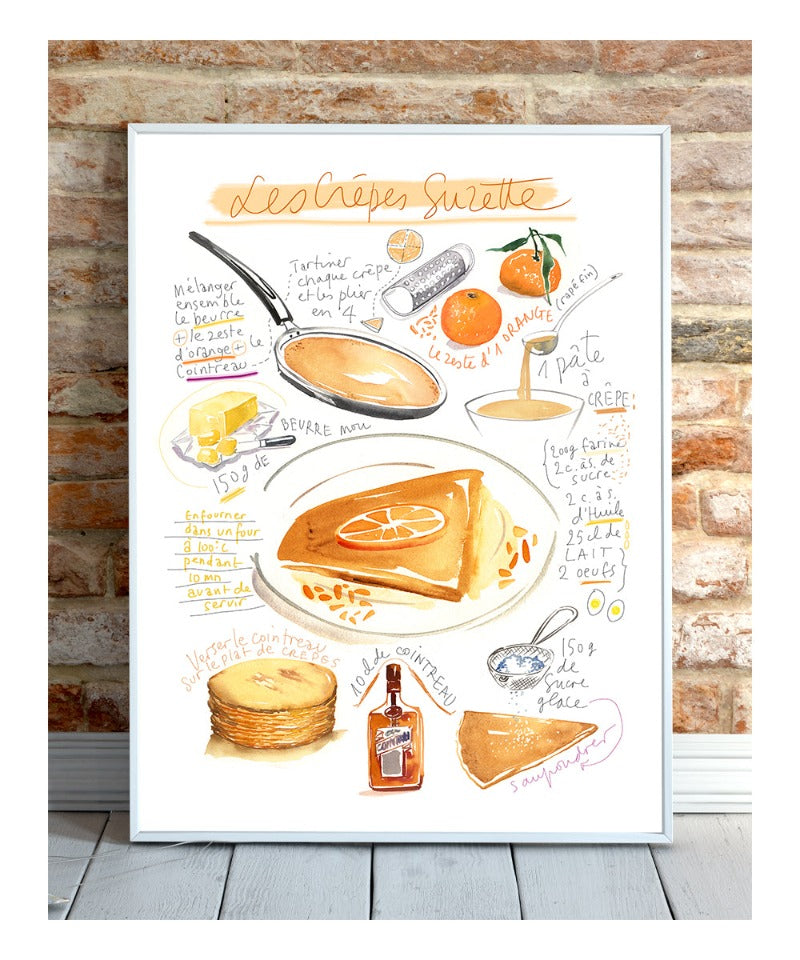The image is a color photograph, taken in portrait orientation, depicting a framed poster or wall art leaning against an older brick wall with tones of red, gray, and cream. The floor beneath is made of vertically oriented gray laminate floorboards. The narrow frame of the poster is silver or gray. The handwritten heading at the top reads "Les Crepes Suzette," with a slight orange brushstroke across the words. The central focus of the poster is a hand-drawn, triangular crepe on a round plate, adorned with a slice of orange. Surrounding the crepe are various illustrated cooking elements: a large skillet on the top left, a stick of butter with a butter knife below it, and two small oranges with green leaves. There's also a white bowl containing a creamy mixture, likely a paté, with a label spooning from it. At the bottom left, there's a stack of crepes and a bottle of liquid. The poster combines cartoonish hand-drawn elements with watercolor effects, giving it an artistic, instructional appearance, possibly explaining how to make the dish in French. The detailed drawing style adds a realistic touch to this decorative piece of cafe or restaurant wall art.